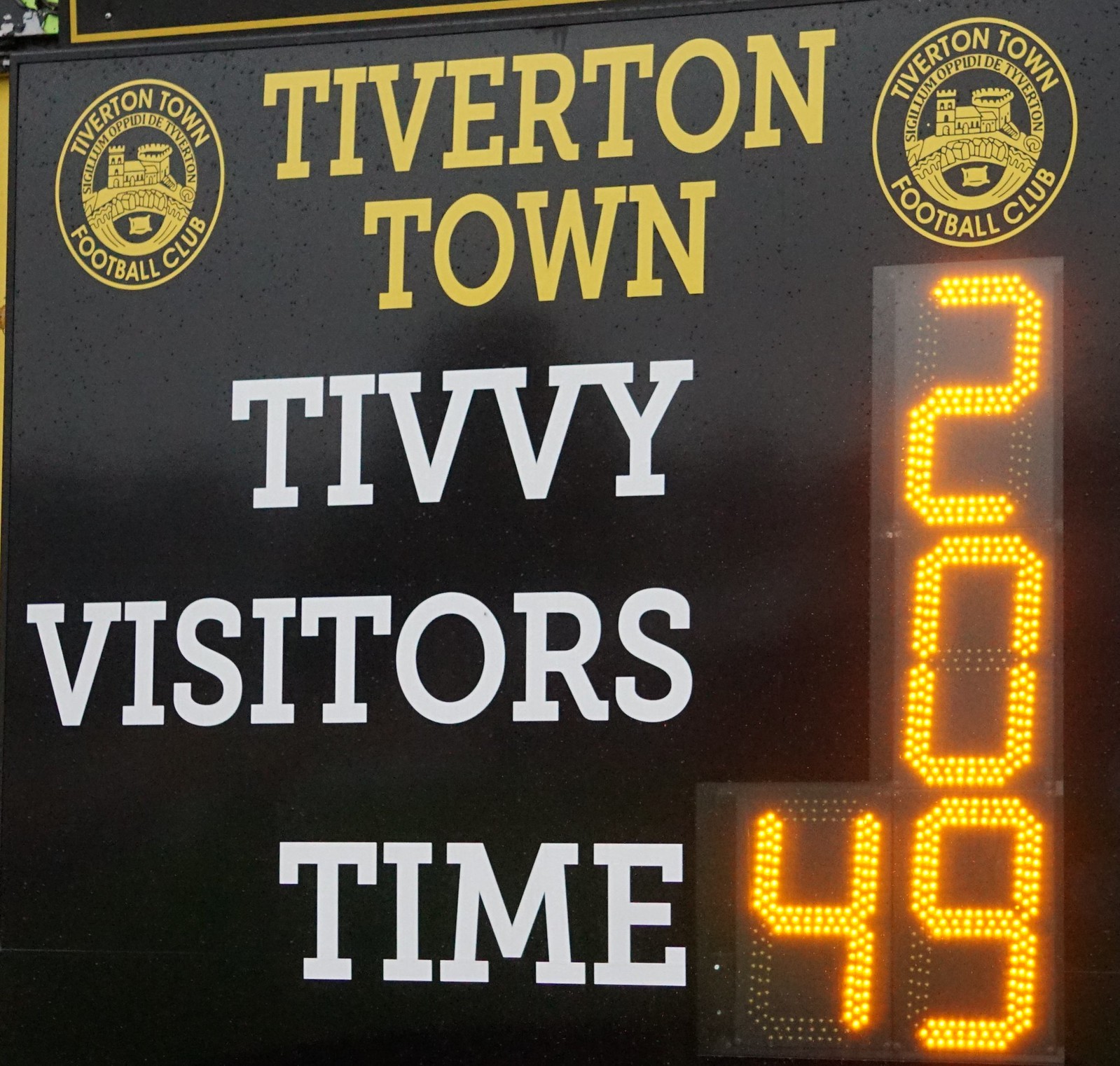The photograph captures a black sports billboard prominently displaying a scoreboard for Tiverton Town Football Club. The top left and right corners feature circular emblems with dark yellow borders, each containing the name "Tiverton Town Football Club" and an illustration resembling a castle. Centered between these emblems, the text "TIVERTON TOWN" appears in an all-caps, serif yellow font. Below this, the scoreboard reads "TIVI" in white, all-caps letters, followed by "VISITORS" and "TIME." Adjacent to these labels, a digital display shows the home team "TIVI" with a score of 2, the visitors with a score of 0, and the time at 49 minutes, all in gold digital numbers. The entire layout of the text and numbers is concise and in all caps.